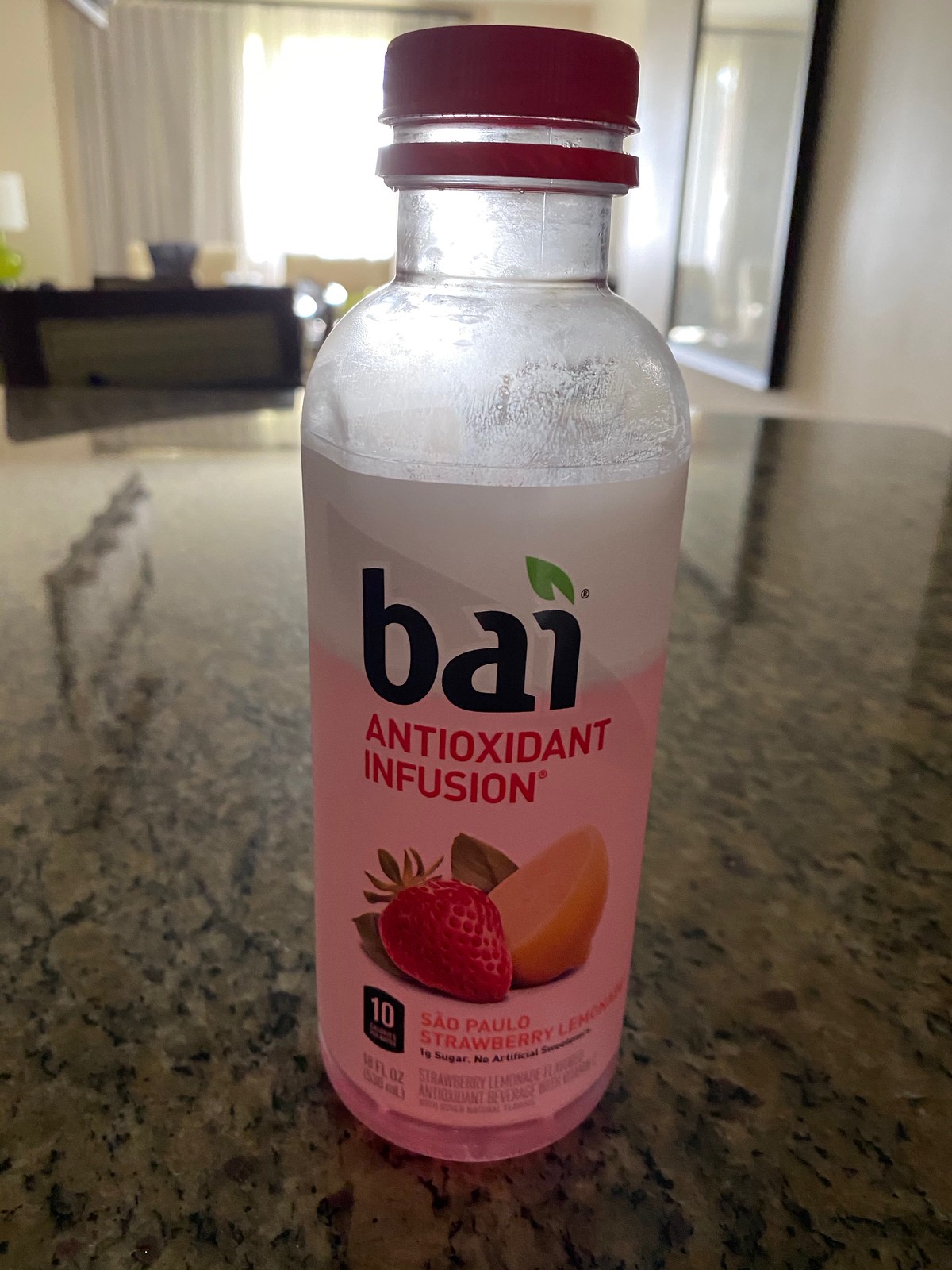The image features a bottle of Bai, with "Bai" spelled out in bold black letters as B-A-I. This is an antioxidant infusion drink. The bottle rests on a multicolored marble table, likely located in a dining room. The background reveals a white wall adorned with a framed picture encased in glass. Additionally, a brown table is visible behind the marble one. Natural brightness streams through a window, suggesting a sunny day outside. Light-colored curtains hang gracefully from the window, further brightening the scene.